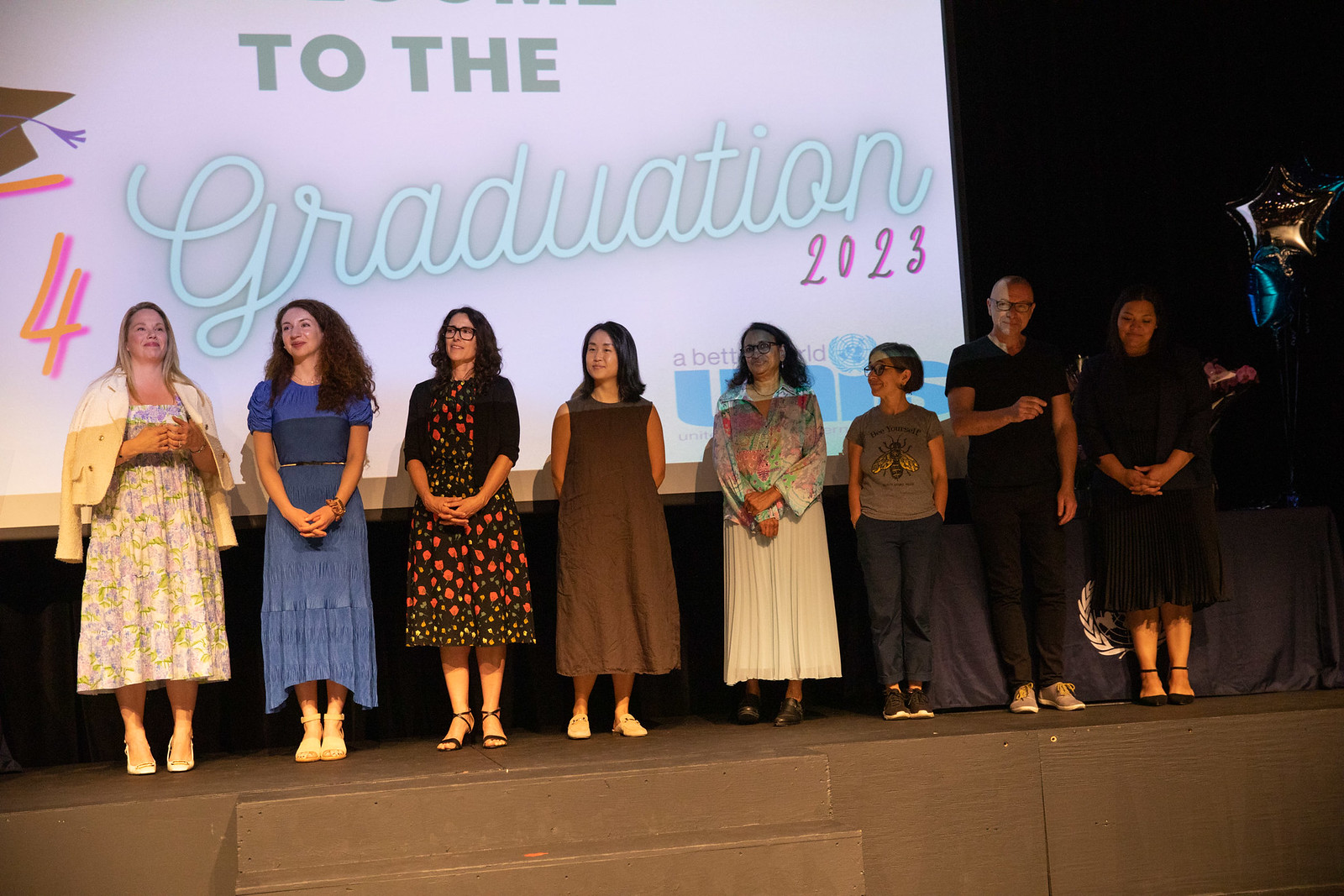This photograph captures a celebratory moment at a graduation ceremony in 2023. Eight individuals, predominantly women with one man and one child, are gathered on a wooden stage painted dark brown, which has steps at the front. The attendees are dressed in a mix of colorful dresses and casual attire, including pants and t-shirts. Behind them, a white screen prominently displays the message "to the graduation 2023," with the word "graduation" styled in a light tealish blue hue, indicative of an Instagram filter. The letter "G" in "graduation" is creatively altered, featuring an orange number four with a hot pink drop shadow. To the right atop the tabled covered with a blue cloth and white emblem, a silver star-shaped balloon adds a festive touch against the black backdrop. Although the specifics of the institution or the level of education aren't clear, the high-quality image captures a moment of joy and achievement, likely celebrating an important academic milestone or special program completion.